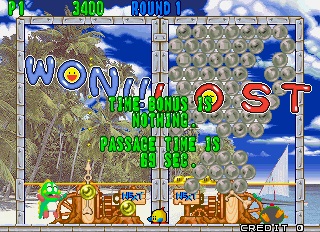This is a detailed screenshot from a Sega Saturn game, "Bust a Move," also known as "Puzzle Bobble." The left side of the screen features a victorious green dinosaur, resembling a turtle, which appears to be smiling. This dinosaur has won the first round, indicated by green bubble letters stating "Round One" at the top and "P1" with a score of "3400." The right-hand side of the screen, displaying the word "Lost" in green bubble letters, is cluttered with numerous gray bubbles, explaining the defeat of the right-side player.

In the center of the screen, it reads "Time Bonus: Nothing" and "Passage Time: 69 Seconds" in green bubble letters. There's a whimsical touch with the letter "O" featuring a smiley face. The background sets a beach scene with palm trees, a sailboat, and a serene ocean, further immersing in the game's playful atmosphere. At the bottom of the screen, it states "Credit: Zero."

Visible on the left side is a contraption with a yellow bubble ready to be launched. The right player’s contraption has a red and yellow bubble, but their screen is almost entirely filled with gray bubbles. This image effectively captures the fun, competitive nature of the game.